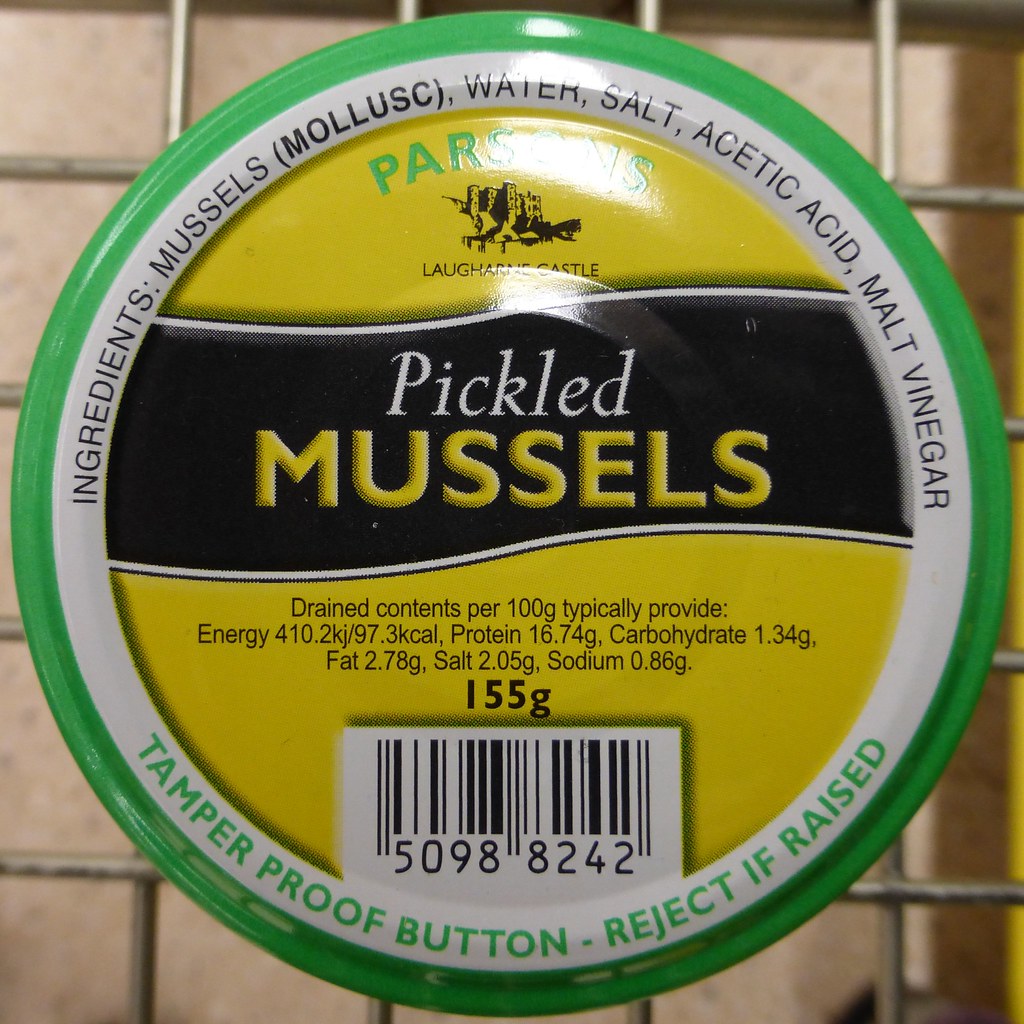The photograph showcases a metallic circular jar lid with a detailed design and multiple inscriptions. The outer edge is accented by a green border, followed by a white border. Within the white border, the top segment bears black text detailing the ingredients: mussels, musk, water, salt, acetic acid, and malt vinegar. In contrast, the bottom part of the white border features green text reading "tamper-proof button, reject if raised." The center of the lid is dominated by a yellow circle that includes various inscriptions. At the top of this circle, green text spells out "Parsons," followed by "Lafarne Castle" in black text. A black banner runs horizontally across the yellow circle, displaying the words "pickled" in white and "mussels" in yellow text. Additional nutritional information is included, although some text may be obstructed by light; it typically indicates that drained liquid per 100 grams provides energy of 410 kJ, 16.74 grams of protein, 1.34 grams of carbohydrates, 2.78 grams of fat, 2.05 grams of salt, and 0.86 grams of sodium. The bottom of the yellow circle also houses a barcode, numbered 50988242.